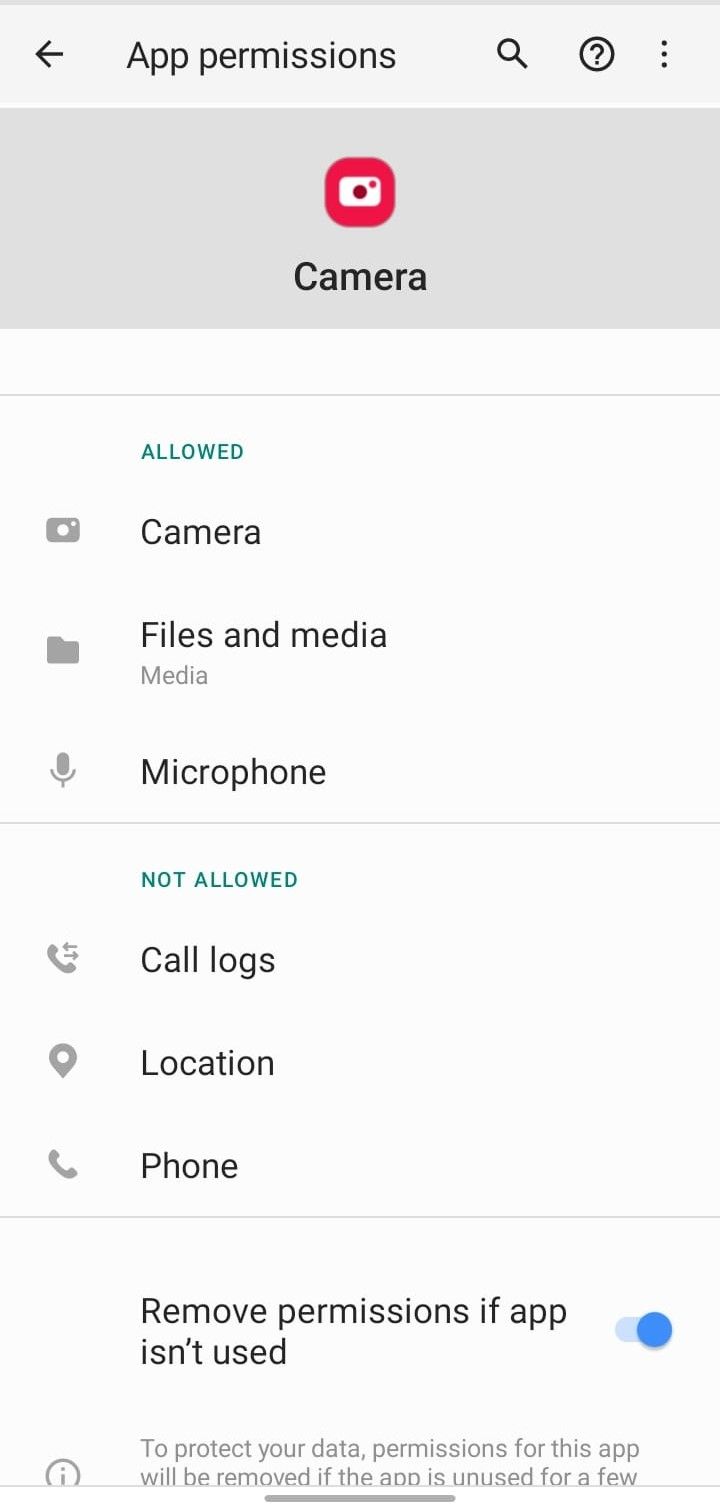The image depicts the app permissions page for a camera setting on a cell phone. In the upper left-hand corner, there is a black back arrow pointing to the left. Next to it, moving right, there is a space, followed by the heading "App Permissions" in black font. Adjacent to this heading on the right, there is a magnifying glass icon, a circle with a question mark inside, and three vertical dots.

Below this heading is a grey box containing a camera icon with the word "Camera" beneath it.

Following this grey box, a section labeled "Allowed" lists the permissions granted to the app. The permissions include:

1. Camera 
2. Files and media (labeled "Media" in smaller, grey font beneath it)
3. Microphone

Further down, a section labeled "Not Allowed" includes:

1. Call logs
2. Location
3. Phone

At the very bottom, there is an option titled "Remove permissions if app isn't used," which is toggled on.